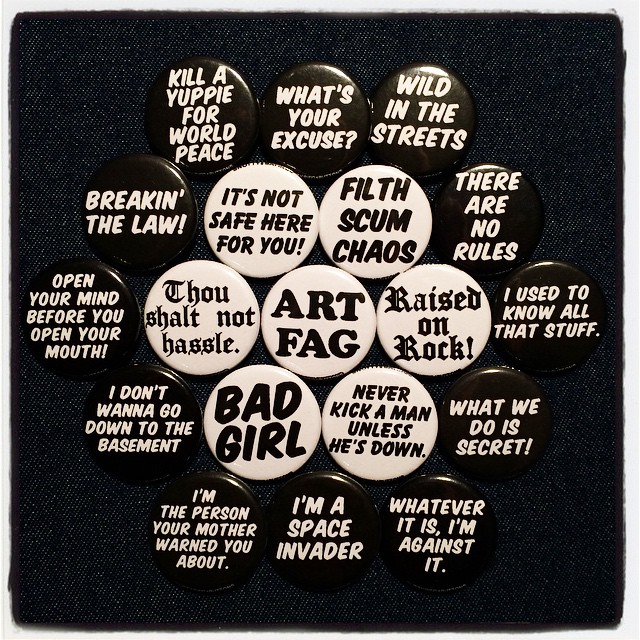In the image, there is a collection of vintage punk rock-style buttons, arranged in a unique and detailed configuration. At the core of this arrangement are seven white buttons forming a hexagonal pattern, with six buttons encircling a central one. Each of these white buttons bears distinct, provocative phrases: "Art Fag" in the center, followed clockwise by "Filth Scum Chaos," "Raised on Rock," "Never Kick a Man Unless He's Down," "Bad Girl," "Thou Shalt Not Hassle," and "It's Not Safe Here for You."

Surrounding this central cluster is a ring of twelve black buttons with white text, further enhancing the rebellious and anti-authoritarian theme. Starting from the top of this outer circle and moving clockwise, the black buttons read: "What's Your Excuse?", "Wild in the Streets," "There Are No Rules," "I Used to Know All That Stuff," "What We Do Is Secret," "Whatever It Is, I'm Against It," "I'm a Space Invader," "I'm the Person Your Mother Warned You About," "I Don't Want to Go Down to the Basement," "Open Your Mind Before You Open Your Mouth," "Breaking the Law," and "Kill a Yuppie for World Peace."

These buttons collectively convey a distinct punk rock ethos, characterized by anti-establishment sentiments and cultural critiques, capturing the rebellious spirit of the 1970s punk movement.